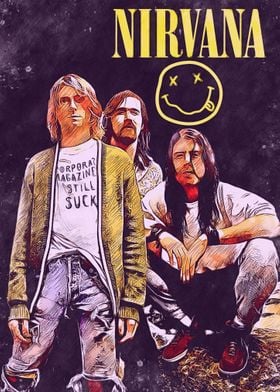The image is an early 90s poster of the rock band Nirvana, featuring a detailed artistic rendition against a black background with white specks resembling stars. At the top, the band name "NIRVANA" is prominently displayed in thick yellow capital letters, stretching from just left of center to the right edge. Below this, a smiley face with crossed-out eyes and a wide, wiggly mouth with a tongue sticking out on the right side adds a quirky element.

In the foreground, the three band members are positioned prominently. Kurt Cobain stands slightly to the left, wearing an open yellow-green jacket over a t-shirt with the partially visible slogan, "Corporate Magazines Still Suck," semi-tucked into his tattered, ripped jeans. His long hair falls just above his shoulders. Dave Grohl, identified by his dark brown shoulder-length hair, stands next to Kurt, partially obscured. Chris Novoselic is squatting on a rock, wearing a white shirt with rolled-up sleeves and dirty black jeans, his long blackish-brown hair reaching his chest. All three members are gazing directly at the viewer, adding to the poster's engaging composition.